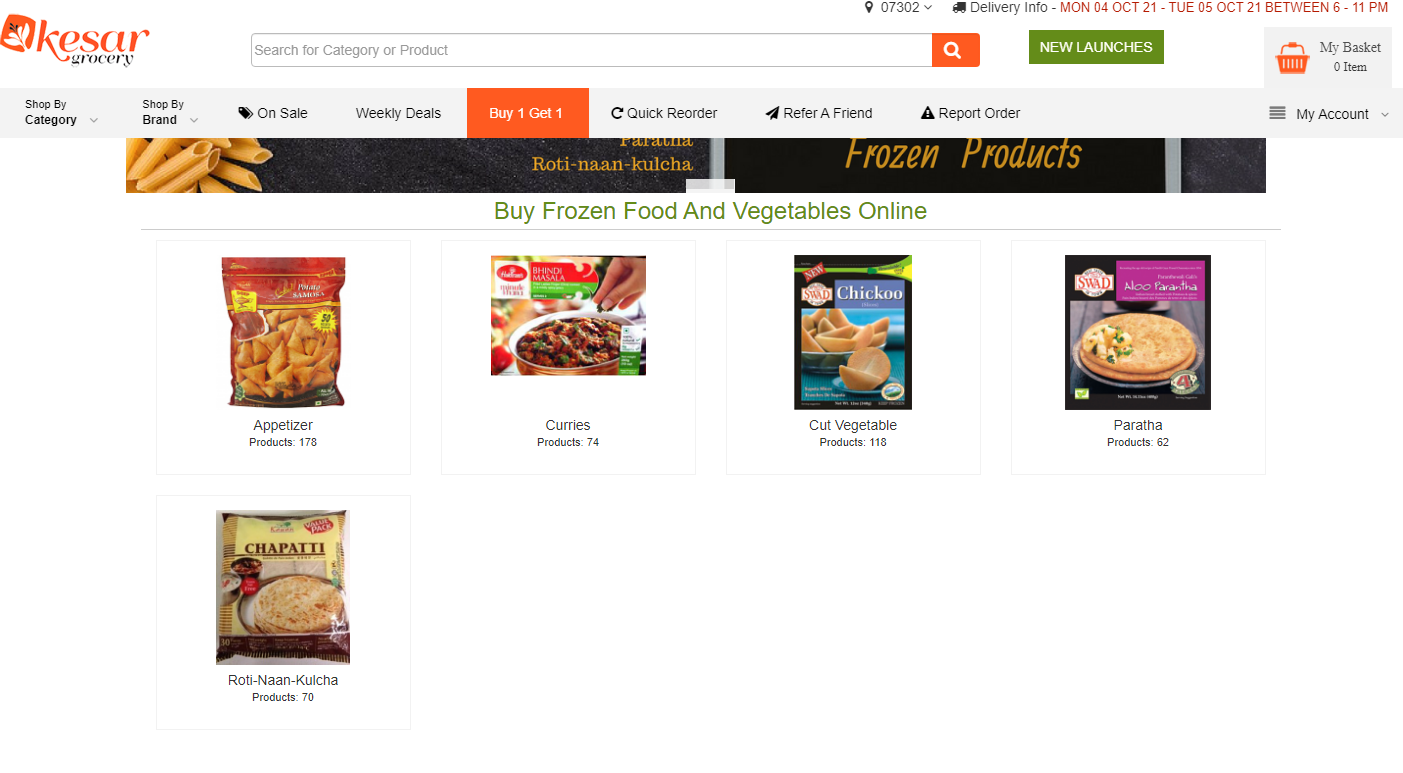The screenshot captures a detailed view of a website belonging to an online grocery store named Kesar Grocery. The layout of the site is in landscape format and features a primarily white background with various images and text elements. In the upper left-hand corner, the Kesar Grocery logo, which appears to incorporate a plant motif, is prominently displayed. 

At the very top center of the page is a search bar for easy navigation, flanked to the right by a link labeled "New Launches" in green. Further right, there is an icon of a shopping basket accompanied by the text "My Basket, zero items." Above this section, you can find additional information about delivery, specifying the address details and delivery times, which state: Monday, October 21st to Tuesday, October 21st, between 6 and 11.

Directly below this, a navigational bar offers various options: "Shop by Category," "Shop by Brand," "On Sale," "Weekly Deals," and in red, "Buy One, Get One." The bar transitions back to a gray base color and includes additional options like "Quick Order," "Refer a Friend," "Report Order," and "My Account" on the furthest right.

Beneath the navigation bar are images of various grocery items including pasta and frozen products. Below this section are additional images featuring categories of frozen fruits, foods, and vegetables. Visible categories include appetizers, curries, cut vegetables, paratha, and roti/naan/kulcha. 

The bottom and right portions of the screen are filled with white, empty space, contributing to a clean, uncluttered look. Overall, the interface presents a standard, straightforward catalog appearance, facilitating easy navigation and shopping for users.